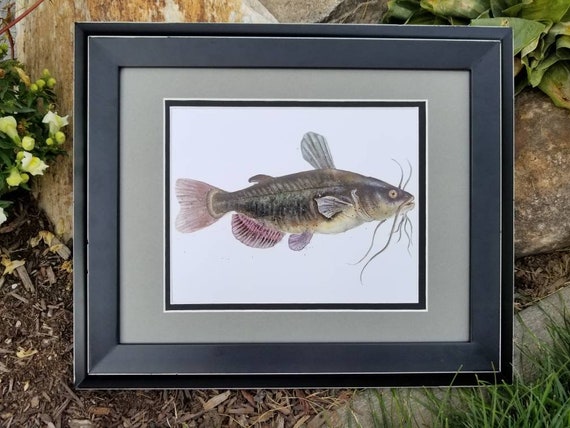The image showcases a detailed and intricately framed portrait of a greenish fish, possibly a catfish or bass, distinguished by its long whiskers and vivid, multicolored fins, including pink-hued dorsal and tail fins. The fish, depicted against a plain white background, features a palette of green, light green, gray, and black. The framing of the portrait is notably complex: a central black border is surrounded by a small white border, followed by a light green mat, and encapsulated in a double gray frame. The entire arrangement is placed outdoors, lying on a bed of mulch, and set against a backdrop of rocks, green grass, some yellow flowers, and other greenery. The composition highlights the fish as the main focus, with the mixture of natural elements around it adding texture and context to the scene.